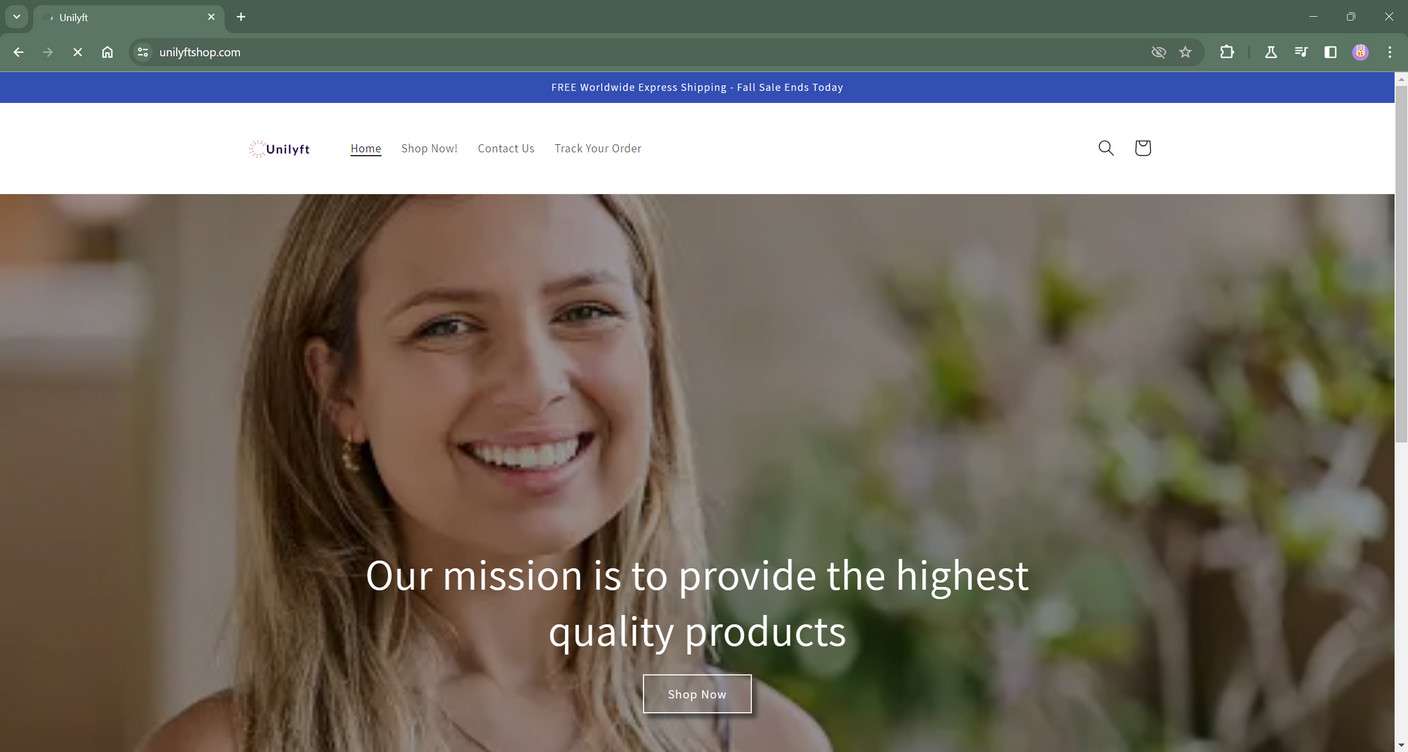A Chrome browser window is open, displaying a webpage for an online store named "Unilift." The browser's theme is customized with a forest green color, affecting the navigation bars but not the website's content. The webpage itself has a blue header that reads "Free worldwide express shipping, fall sale ends today," which transitions into a predominantly white background. 

The top navigation menu includes options such as "Home," "Shop Now," "Contact Us," and "Track Your Order." Dominating the central area of the page is a stock photo of a young white woman, smiling warmly in an office-like setting. The background behind her includes a shrub or plant near a white wall, suggesting the space is open and well-lit. Above the image, there is a mission statement reading, "Our mission is to provide the highest quality products," accompanied by a "Shop Now" button. The specific products sold by Unilift are not clearly indicated on this particular page.